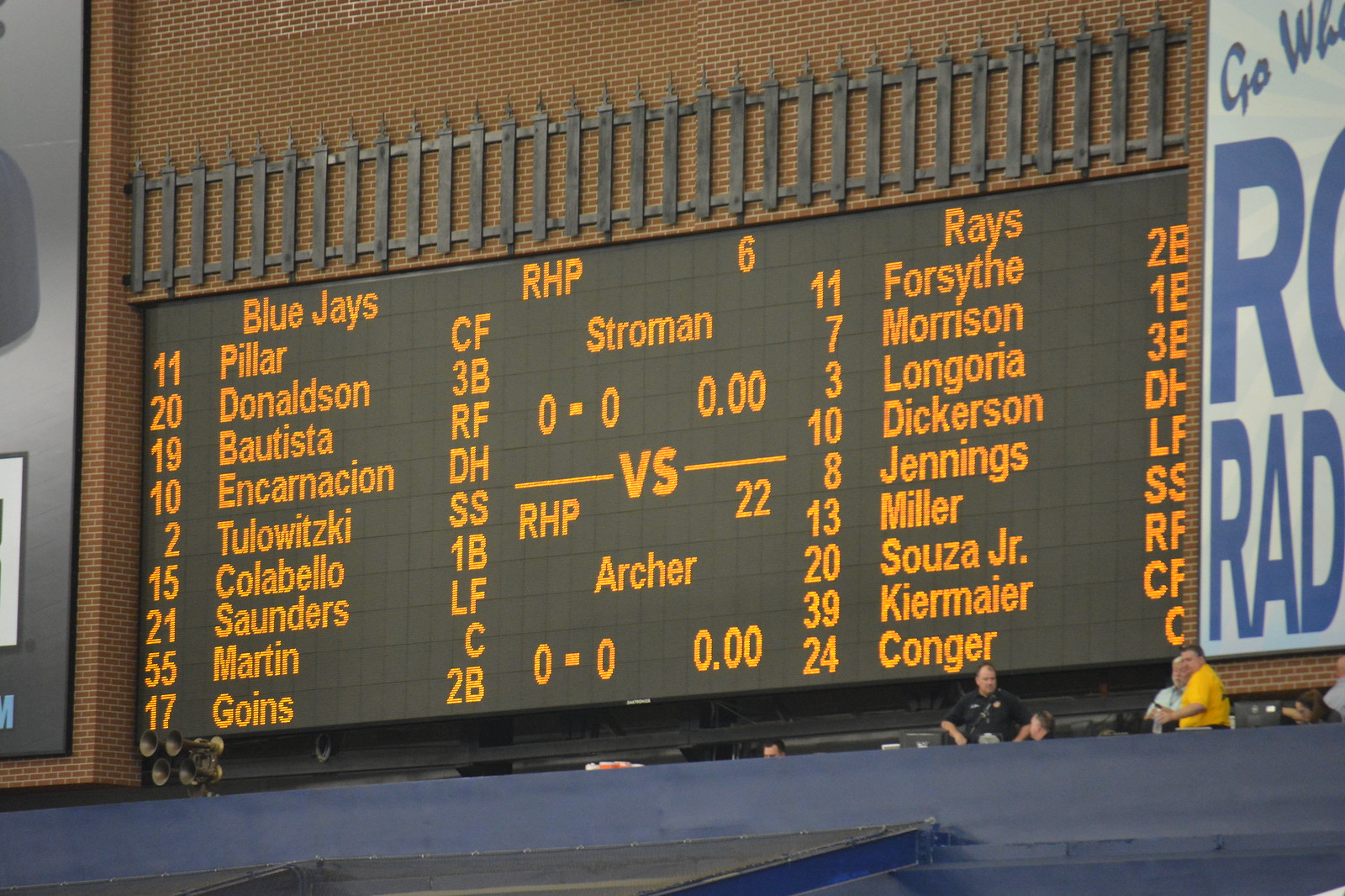The image shows an expansive digital scoreboard attached to the side of a brick wall building, creating a stark contrast that highlights its electronic brightness against the traditional structure. The scoreboard prominently displays the lineup for a baseball game between the Toronto Blue Jays and the Tampa Bay Rays, with the lettering illuminated in bold orange against a black background.

In the left column, underneath the Blue Jays' header, the players’ details are listed, including:
- Kevin Pillar (CF, #11), 
- Josh Donaldson (3B, #20),
- Jose Bautista (RF, #19),
- Edwin Encarnacion (DH, #10),
- Troy Tulowitzki (SS, #2),
- Chris Colabello (1B, #15).

The right column displays the Tampa Bay Rays lineup:
- Logan Forsythe (2B),
- Logan Morrison (1B),
- Evan Longoria (3B),
- Corey Dickerson (LF),
- Desmond Jennings (RF),
- Brad Miller (SS),
- Steven Souza Jr. (CF),
- Kevin Kiermaier (CF),
- Hank Conger (C).

Additional details indicate the presence of the starting pitchers—Marcus Stroman for the Blue Jays and Chris Archer for the Rays—featured prominently in the center of the board. The players, dwarfed by the sheer size of the scoreboard, are visible at the bottom, illustrating the scope of the display and adding to the sense of grandeur.